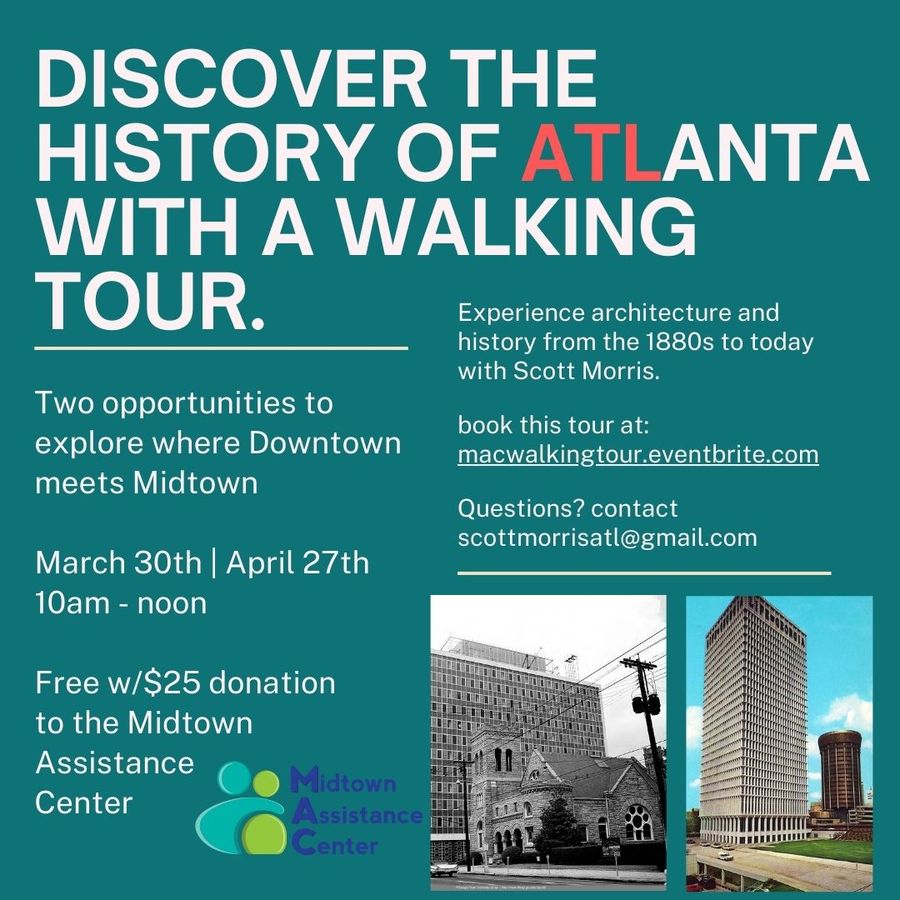The advertisement features a vibrant green background with large white text at the top that reads, "Discover the History of Atlanta with a Walking Tour." Below this heading, there's an underlined subtitle stating, "Two opportunities to explore where downtown meets midtown: March 30th, April 27th, 10 a.m. to noon. Free with a $25 donation to the Midtown Assistance Center." 

On the left side, under the subtitle, a logo of the Midtown Assistance Center depicts two human figures hugging, one in green and one in yellow. To the right, additional text invites participants to "Experience architecture and history from the 1880s to today with Scott Morris." It also provides booking details at "packwalkingtour.eventbrite.com" and contact information via "scottmorrisatl@gmail.com."

At the bottom of the poster, there are two images representing Atlanta's architectural history: an old photograph showing a vintage building with a road, electric poles, and a vintage car, and a modern vibrant image of a tall skyscraper with a flyover and moving cars against a backdrop of blue sky and white clouds. The juxtaposition of these images underscores Atlanta's historical evolution from past to present.